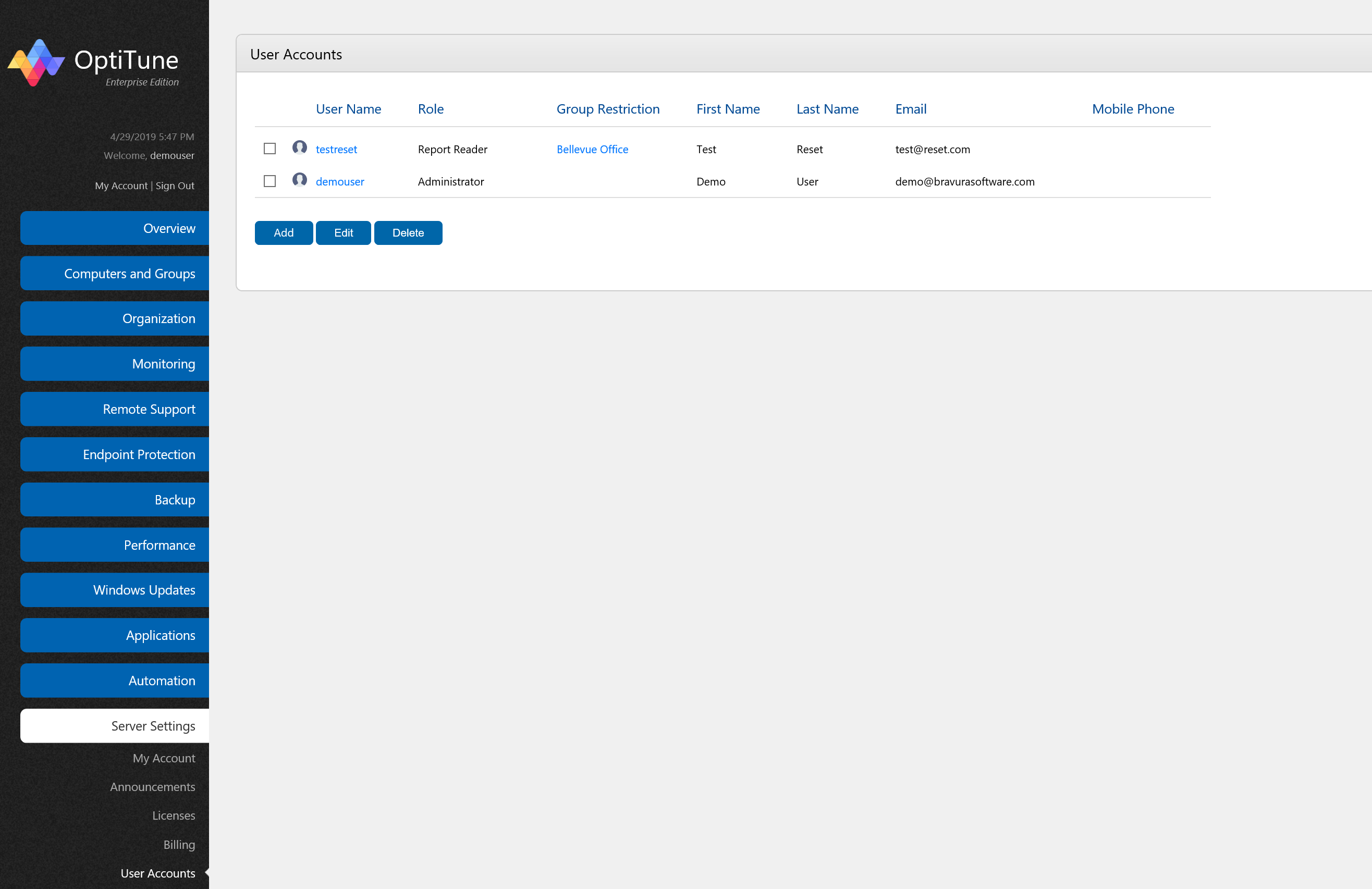This is a screenshot of a website featuring a structured interface. On the left side, there is a vertical black sidebar. At the top of this sidebar is a colorful logo resembling a rainbow splash, accompanied by the text "OptiTune" in white font. Beneath the logo, there is smaller white text that is difficult to read. The sidebar contains several options listed in blue rectangles with white font: Overview, Computers and Groups, Organization, Monitoring, Remote Support, Endpoint Protection, Backup, Performance, Windows Updates, Applications, Automations, and Server Settings. Further down, additional options in white text include My Account, Announcements, Licenses, Bling, and User Accounts.

On the right side of the screenshot, the main webpage area has a gray background. At the top, in black font, it reads "User Accounts." Below this heading is a white rectangular section. Within this section, headings in dark blue font label different fields: Username, Role, Group Restriction, First Name, Last Name, Email, and Mobile Phone.